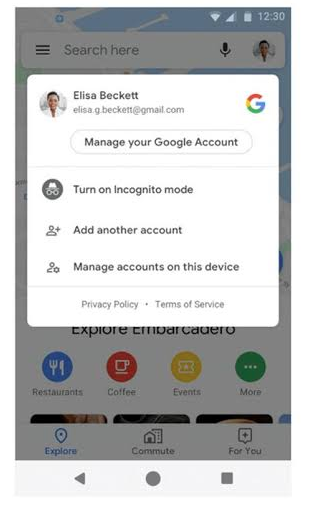**Caption:**

This screenshot, taken from a smartphone at 12:30 PM with a mediocre to fair Wi-Fi signal and modest battery usage, captures a Google search in the background. Dominating the screen is a prominent pop-up that partially obscures the search results. The pop-up displays various account management options for the user, Alicia Lisa Beckett, whose email is GBeckett@JML.com. The message includes the option to manage the Google account associated with the email ElisaGBeckett@gmail.com. A white rectangular box offers the option to "Turn on Incognito mode," accompanied by the incognito mode icon— a figure wearing a hat and binoculars. Below this, there are options for adding another account and managing accounts on the current device, marked with a check symbol. At the bottom of the pop-up, links to "Privacy Policy" and "Terms of Service" are visible. Visible through the transparency of the pop-up, the Google search page is faintly discernible, showing elements such as the search bar at the top and various search categories including “Restaurants,” “Coffee,” “Events,” and more.